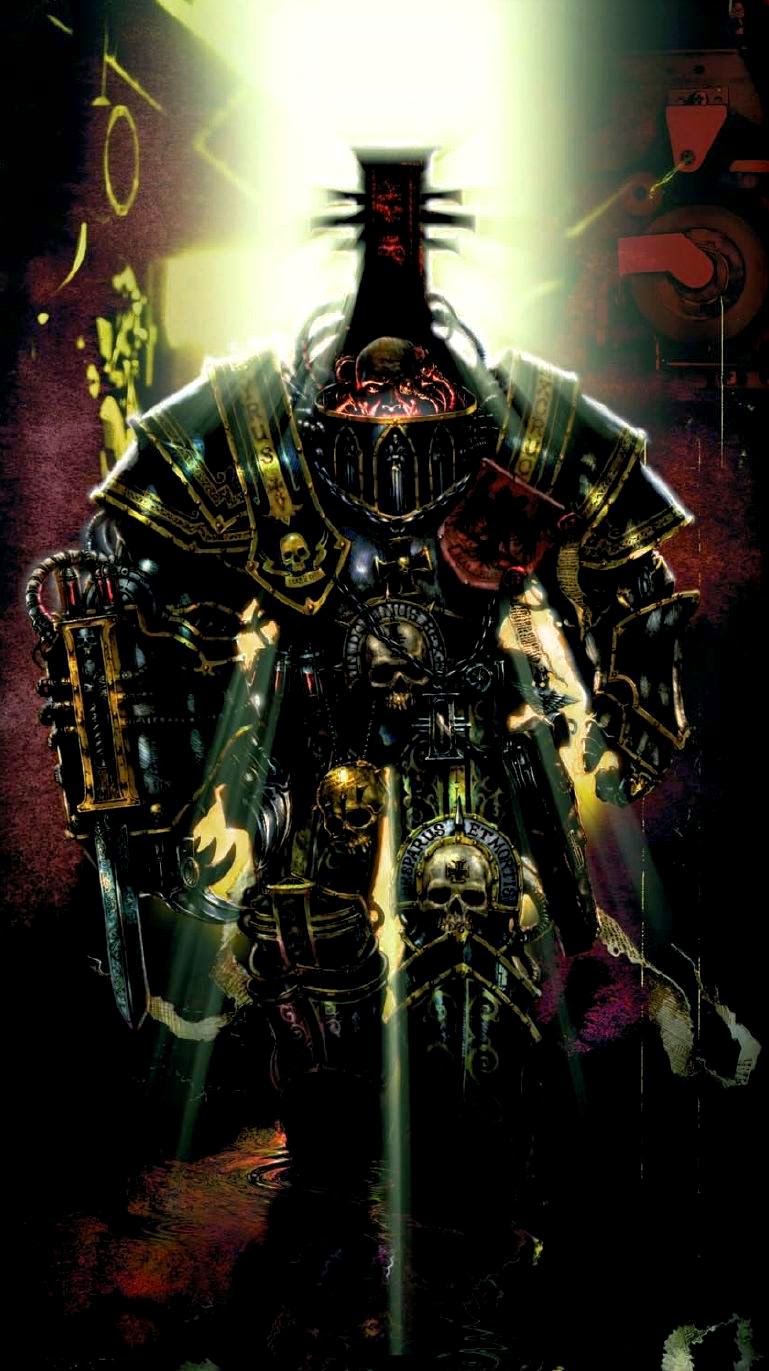In this vivid and intricate color illustration, we see a towering armored warrior, named Tyrus. The character is encased in an over-the-top exoskeletal suit that is heavily adorned with skulls and Latin phrases engraved around them. A unique feature of this suit is a rectangular area jutting out from the top, adorned with a pink glowing light that surrounds it, adding a surreal atmosphere. Surprisingly, the head is not positioned at the top but instead emerges in a diminutive form from where the neck would typically be. Only the top of this head, down to about the nose, is visible through an opening in the armor. The warrior carries an enormous, indiscernible weapon in the right hand, and there is another skull prominently hanging from the waistband. Mechanical contraptions, which include rotor blades and other devices, can be seen protruding from behind this head, contributing to the fantastical and industrial aesthetic. The background is dark and out of focus, featuring indistinct red and purple objects that further emphasize the otherworldly setting. The light in this fantasy image, although surreal and bright, enhances the mystique and illustrative style, ultimately creating a riveting portrayal of Tyrus, the deadliest fictional character in this fantasy realm.